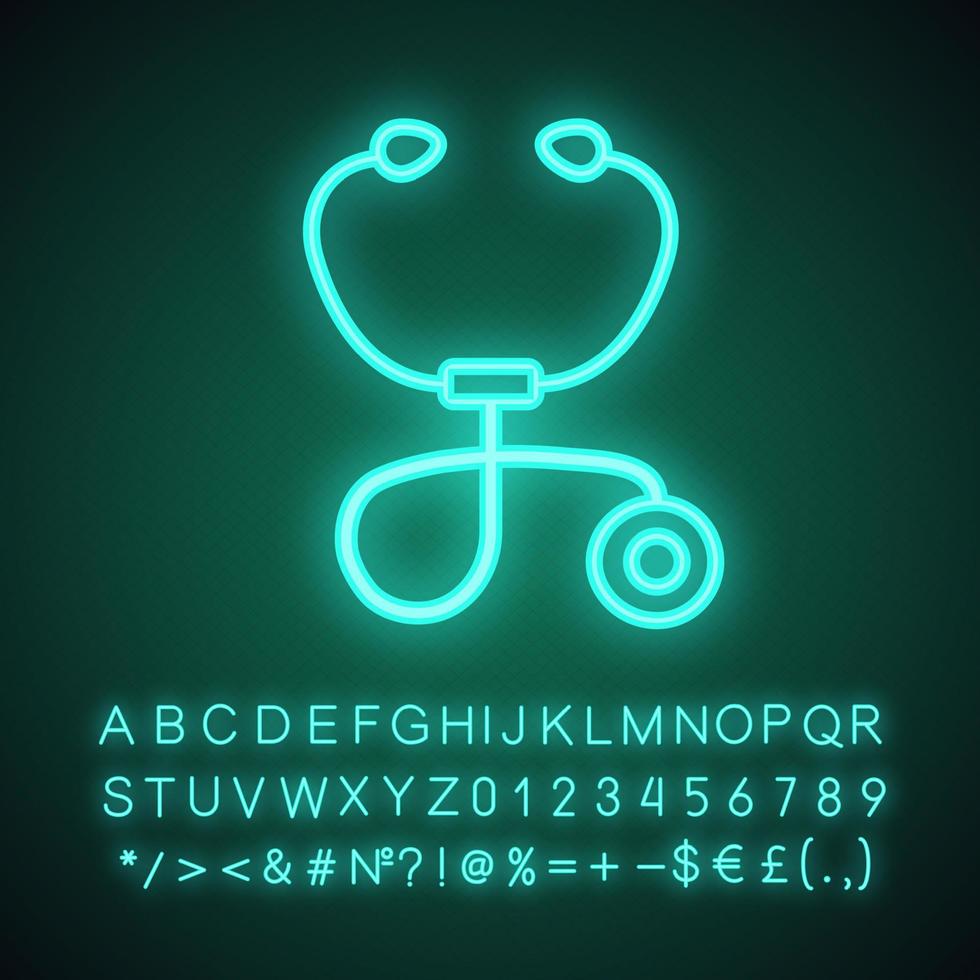A neon, glow-in-the-dark image with a dark teal backdrop fading into black at the corners features the bright teal silhouette of a stethoscope in the center. This stethoscope, possibly a neon lamp, is outlined in a neon greenish-blue hue. It’s a simplistic, artistic representation — with two earbuds, a central rectangle, a looping string leading to the round hearing disc depicted by two concentric rings. Beneath the stethoscope are three lines of glowing text: the complete alphabet in capital letters, the numbers 0 through 9, and an assortment of symbols including asterisk, backslash, forward arrow, back arrow, number sign, question mark, exclamation point, at sign, percent sign, equal sign, plus sign, minus sign, dollar sign, euro sign, British pound sign, parentheses, period, and comma. This square-shaped animated image thus highlights a vibrant and intricate display of a stethoscope with accompanying characters, suggesting it might be an advertisement for a customizable neon lamp.